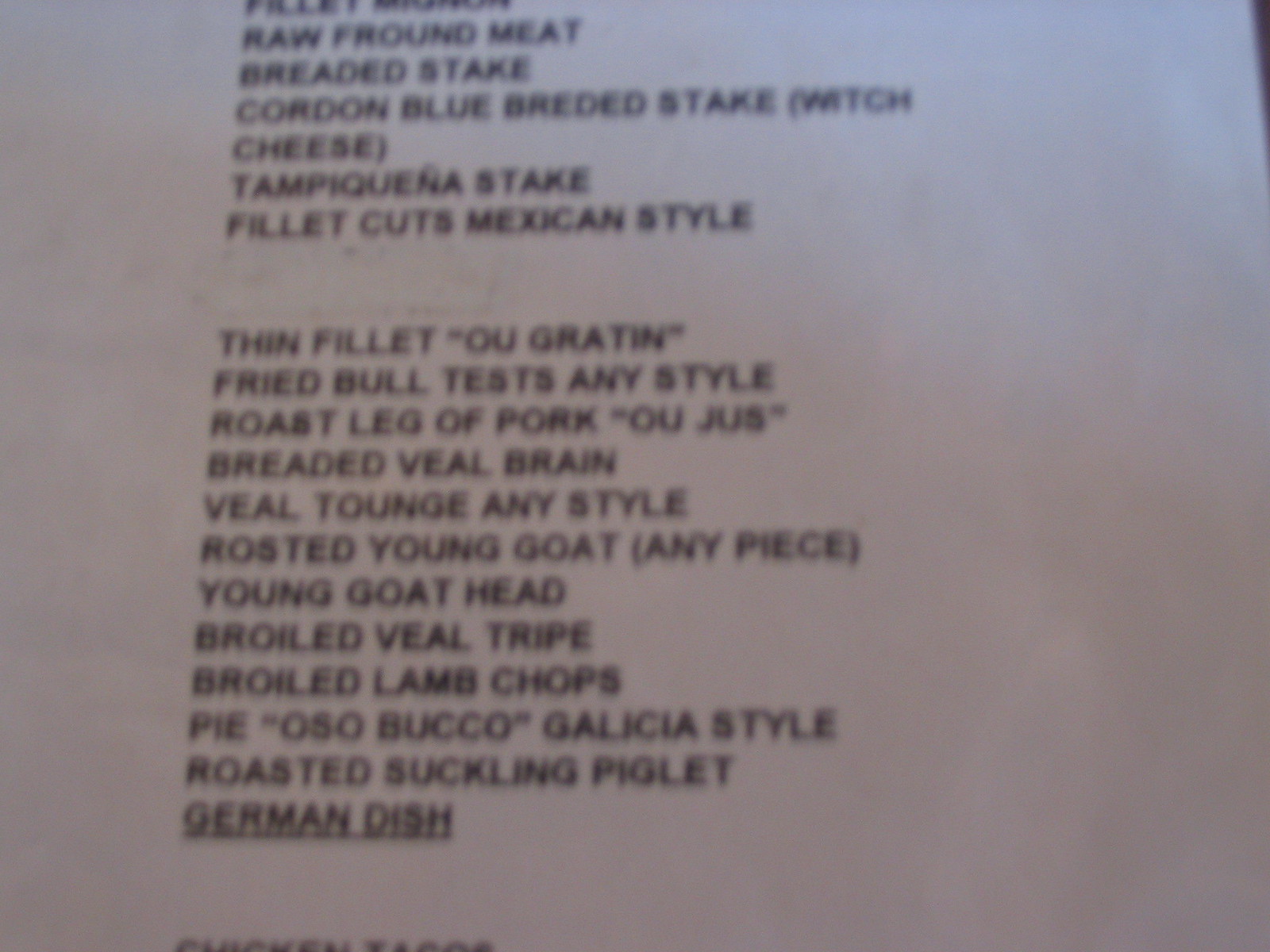This photograph captures a highly out-of-focus image of a white piece of paper containing a handwritten list. The text is extremely faded and difficult to read, revealing numerous misspellings and unique culinary offerings. The list, from the top, includes items such as "Raw Frowned Meat," "Breaded Steak" (misspelled as "S-T-A-K-E"), and "Cordon Bleu" (incorrectly written as "B-R-E-D-E-D S-T-A-K-E"). The content also describes "Watch Cheese," evidencing poor spelling, and continues with "Tampiquenia Steak" (again "S-T-A-K-E") and "Filet Cuts, Mexican Style."

A notable gap separates these from the next section, which lists "Fin Fillet" (spelled with two L's), "Owl-Gratin" (misspelled "O-U-gratin"), and unique dishes like "Fried Bull Testicles, Any Style," presumably referring to testicles. Further down, the list includes "Roast Leg of Pork," oddly paired with "O-Juice" (instead of the correct "Au Jus"). Other intriguing entries are "Breaded Veal Brain," "Veal Tongue, Any Style," "Roast a Young Goat, Any Piece," "Young Goat Head," and "Broiled Veal Tripe," among other items not clearly deciphered due to the blurry and faded quality of the photograph.